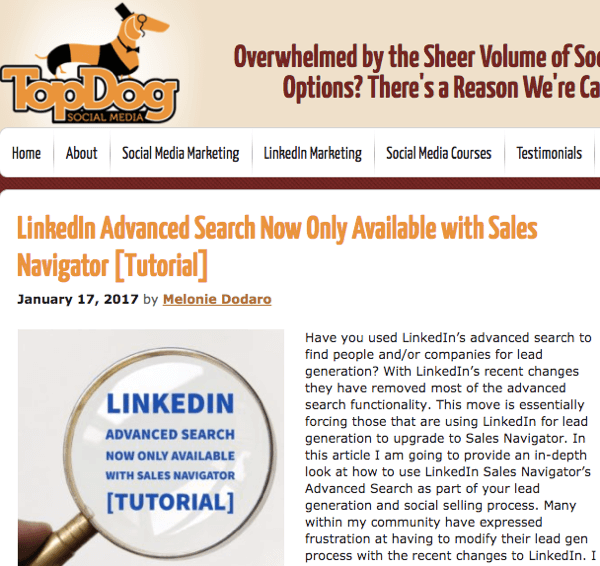Here is the detailed and cleaned-up caption:

---

The website displayed is titled "Top Dog" and prominently features an animated dog as its mascot. At the top, a menu bar includes several options: Home, About, Social Media, Marketing, LinkedIn Marketing, Social Media Courses, Testimonials, and LinkedIn Advanced Search. A special note highlights that the LinkedIn Advanced Search feature is not only available with Sales Navigator. An article dated January 17th by Melinda Dodoro is mentioned, describing a tutorial on using the LinkedIn Advanced Search without Sales Navigator. The image includes an icon of a magnifying glass labeled "LinkedIn Advanced Search, Not Available with Sales Navigator Tutorial." Additionally, a box contains detailed information about these topics, guiding the viewer through the various offerings of the website.

---